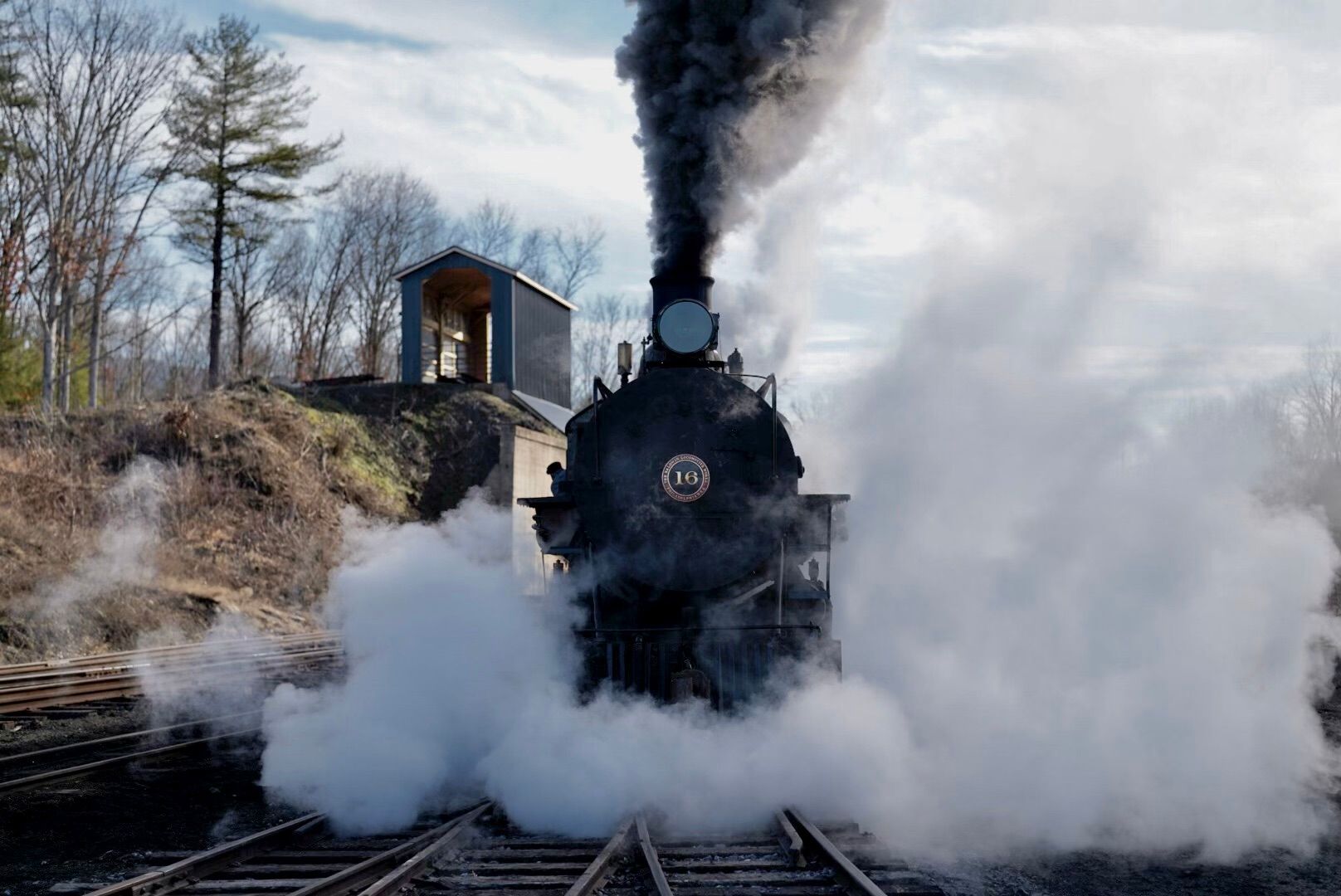The photograph captures an old-fashioned, black steam engine train, emblazoned with the number 16 prominently on its front, chugging towards the viewer along a set of tracks. The powerful locomotive is enveloped in a thick cloud of white steam that billows around its base and sides, while dark smoke pours from its chimney, accentuating its motion. The scene is set outdoors on what appears to be a late fall or winter day, as the barren deciduous trees in the background have lost their leaves. Amidst this natural backdrop, a wooden shed or barn, gray and seemingly doorless, stands to the left of the tracks atop a small hill, with a mix of pine and leafless deciduous trees surrounding it. The sky overhead is mostly cloudy, complementing the overall atmosphere of the image. The vivid, contrasting colors and dynamic elements of steam and smoke make this a compelling and evocative snapshot of industrial history in a seasonal landscape.